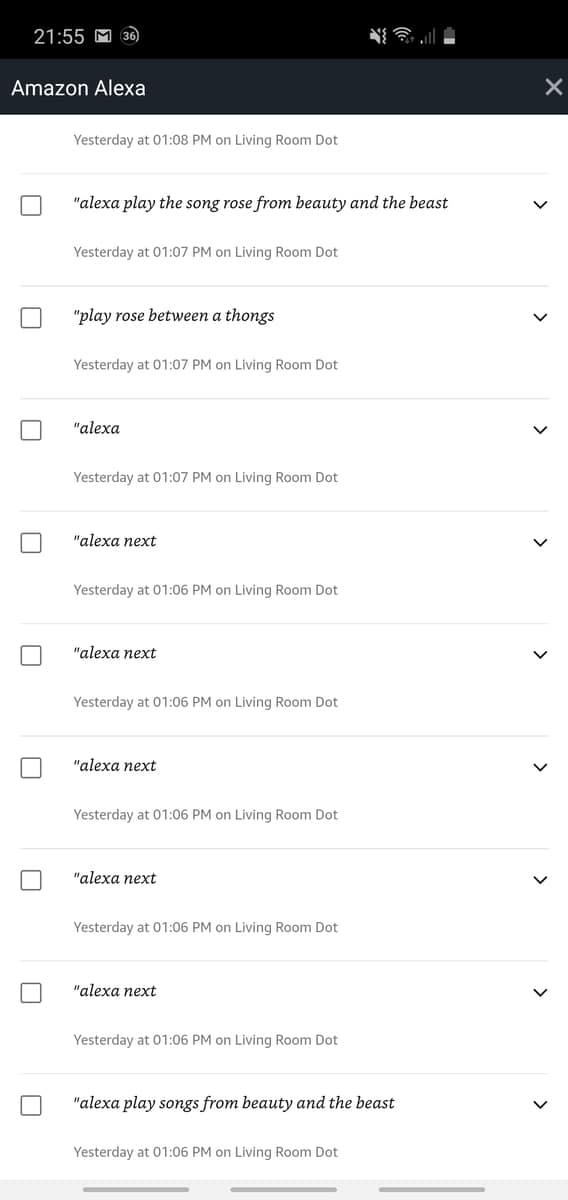Screenshot of an Android device showing the time as 21:55. In the status bar, there is a Gmail icon with the number 36 next to it, indicating unread emails. The volume icon is crossed out, signifying the device is on mute. Wi-Fi signal and service bars are present, along with a low battery indicator.

The screen displays activities from the Amazon Alexa app. At the top, "Amazon Alexa" is shown with a close (X) icon next to it. Below that, it reads "Yesterday at 1:08 PM on Living Room," indicating the time and location of the Alexa activities. There are ten white squares showing different Alexa commands from the previous day:

1. "Alexa, play the song 'Rose' from Beauty and the Beast" – Yesterday at 1:07 PM on Living Room.
2. "Play 'Rose' between a thong" – Yesterday at 1:07 PM on Living Room.
3. "Alexa" – Yesterday at 1:07 PM on Living Room.
4. "Alexa, next" – Yesterday at 1:06 PM on Living Room.
5. "Alexa, next" – Yesterday at 1:06 PM on Living Room.
6. "Alexa, next" – Yesterday at 1:06 PM on Living Room.
7. "Alexa, next" – Yesterday at 1:06 PM on Living Room.
8. "Alexa, play songs from Beauty and the Beast" – Yesterday at 1:06 PM on Living Room.

Each Alexa command is displayed in bold text with quotation marks and has a drop-down arrow next to it for additional options or details.